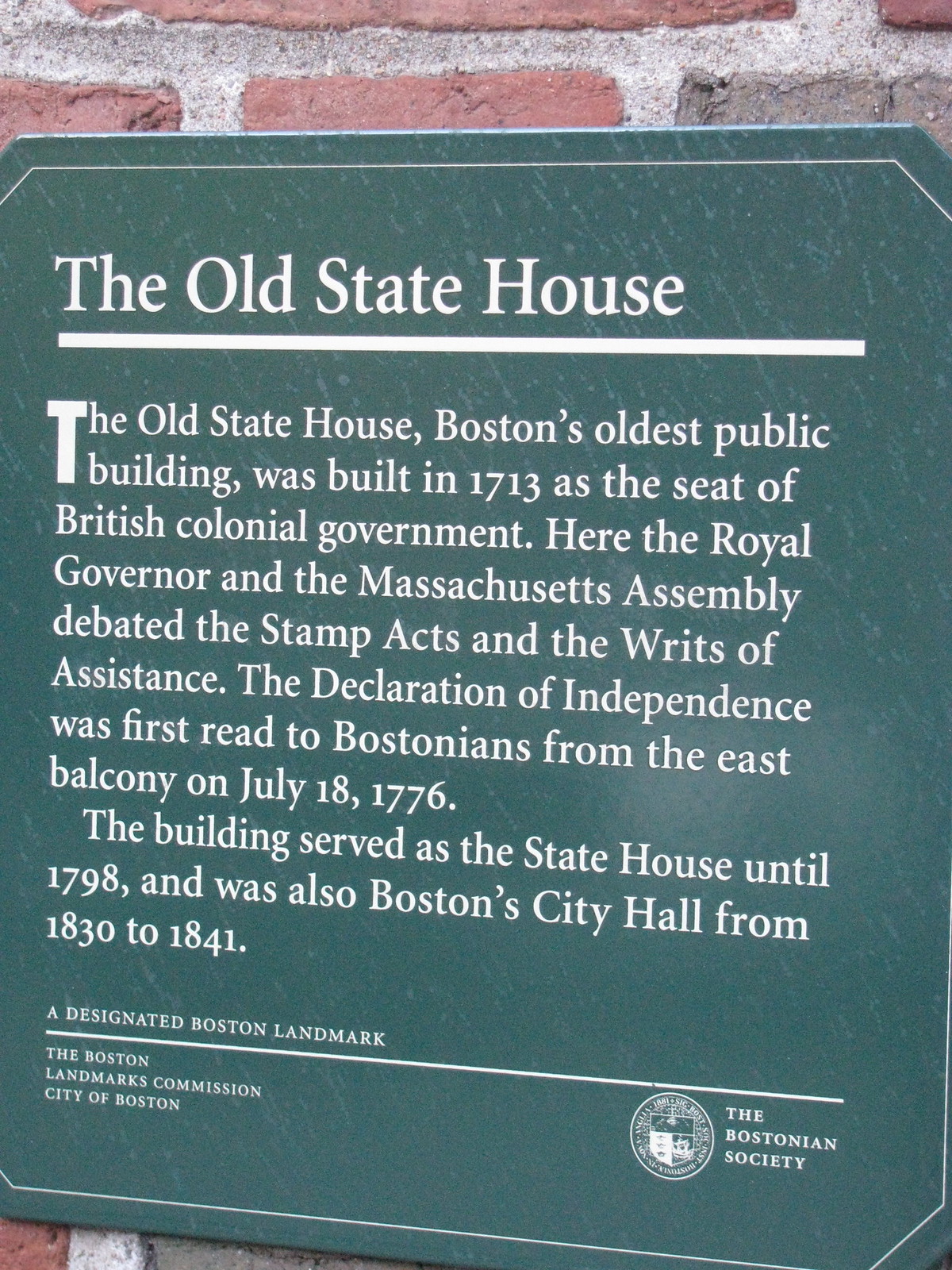The image depicts a green sign affixed to the side of a brick building, bordered by a thin white line. The sign bears the inscription "The Old State House" in white font. Below this, a detailed description reads: "The Old State House, Boston's oldest public building, was built in 1713 as the seat of the British colonial governor. Here, the Royal Governor and the Massachusetts Assembly debated the Stamp Acts and the Writs of Assistance. The Declaration of Independence was first read to Bostonians from the East Balcony on July 18, 1776. The building served as the State House until 1798 and was also Boston's City Hall from 1830 to 1841." At the bottom of the sign is the emblem of the Bostonian Society, signifying its status as a designated Boston landmark by the Boston Landmarks Commission, City of Boston.